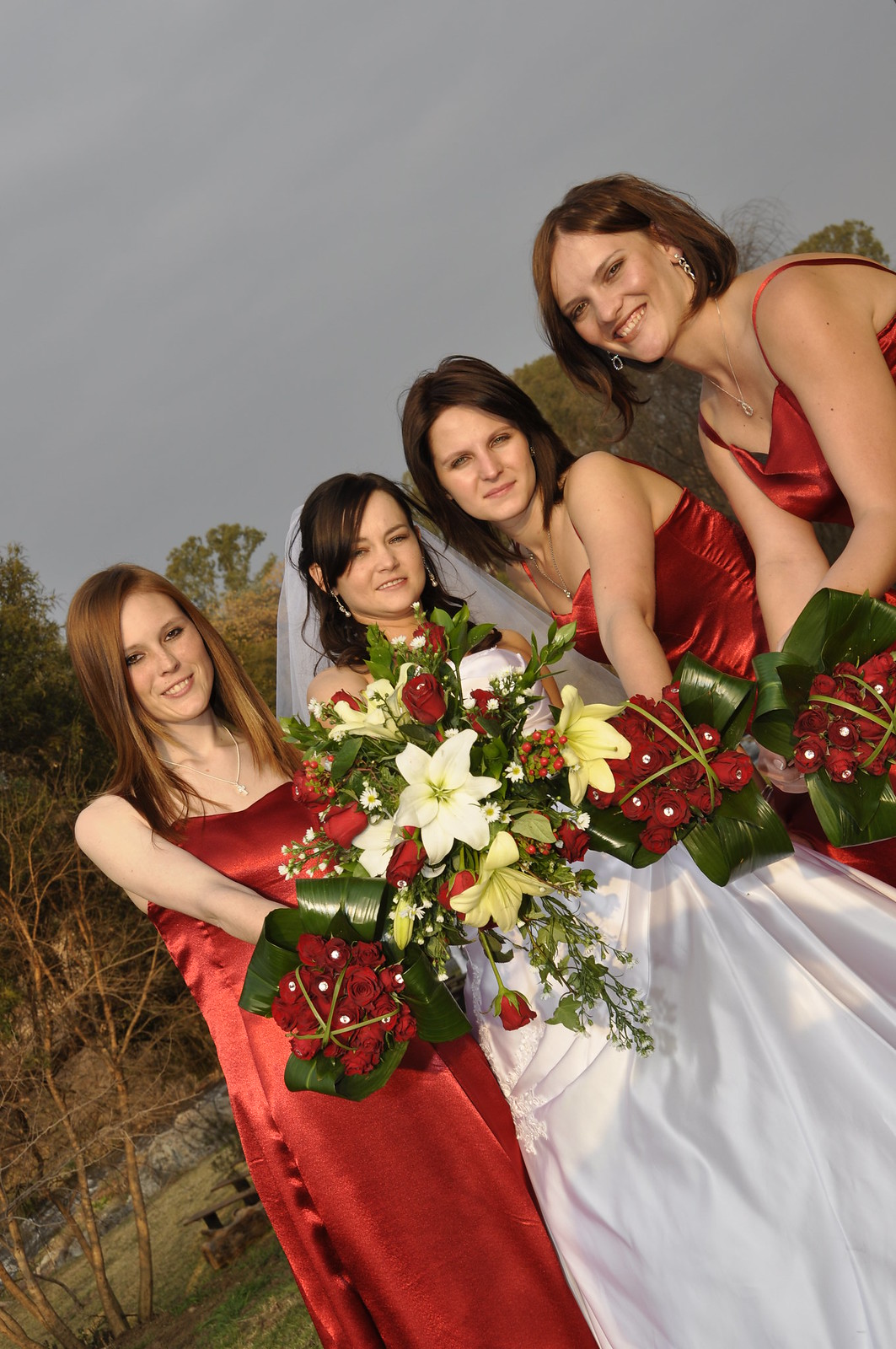This photograph captures a serene outdoor scene of a bride and her three bridesmaids, set against a backdrop of bare trees and a hazy sky. The bride, radiant in a strapless white satin wedding gown, holds an opulent Christmas-themed bouquet featuring large white lilies, red roses, holly berries, and delicate baby's breath, adorned with folded green ribbon details. Her shoulder-length dark hair is partially covered by a veil that drapes down her back. She is flanked by her bridesmaids, each in matching long red satin gowns. They too hold bouquets of red roses, each rose accented with a white pearl at its center.

On the far left stands the first bridesmaid, her straight, shiny shoulder-length hair a striking reddish hue. She wears a necklace with a cross and has brown eyes enhanced by lipstick. Beside her, the second bridesmaid, with shoulder-length dark hair, attentively helps to hold the bride’s bouquet. The third bridesmaid, positioned to the bride’s right, sports chin-length auburn hair and accessorizes with silver or glittery dangly earrings. All three bridesmaids exude joy, their smiles adding warmth to the overcast day.